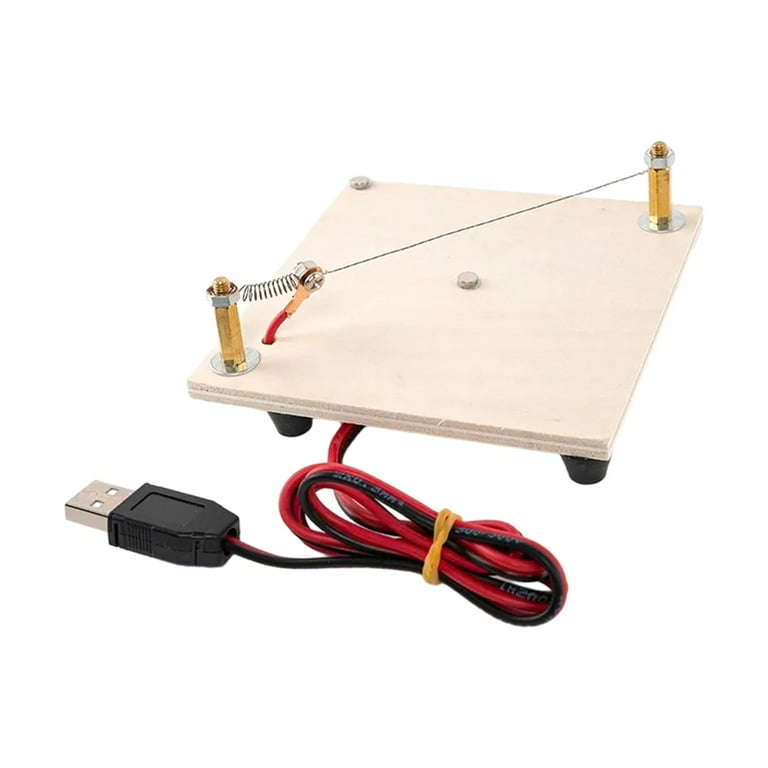The image depicts a science fair project or experimental display featuring a wooden square board with tapered cylindrical black rubber feet. The off-white wooden square serves as the base for the setup. Diagonally positioned from the lower left-hand side to the upper right-hand side of the square are two brass screws fastened with silver metallic nuts and washers. These brass screws are connected by a wire, which is held aloft by the nuts. Below this arrangement, a red and black twisted wire is visible, with the red wire running underneath the wooden base. The wire bundle is secured with a rubber band, and the black wire extends to the left, terminating in a black USB plug.